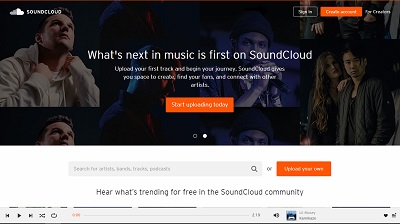Screenshot of the SoundCloud landing page. The top of the image is dominated by a bold text that reads, "What's next in music is first on SoundCloud." Below it, there are options to "Sign in" or "Create account," and a call-to-action encouraging users to "Upload your first track and begin your journey." The page explains that "SoundCloud gives you space to explore, find your fans, and connect with other artists." Additional text urges users to "Start uploading today" and highlights that they can "hear what's trending for free on the SoundCloud community."

The visual elements include pictures of diverse creators: a depressed-looking Asian individual with a transgender woman affectionately hanging on his shoulder, a black male wearing a beanie and holding a microphone, and a young white male in a white hoodie, gripping his collar. The overall color scheme transitions from a black background at the top to white at the bottom, with three prominent orange buttons garnering attention. The design effectively emphasizes SoundCloud's appeal to a diverse community of music creators.